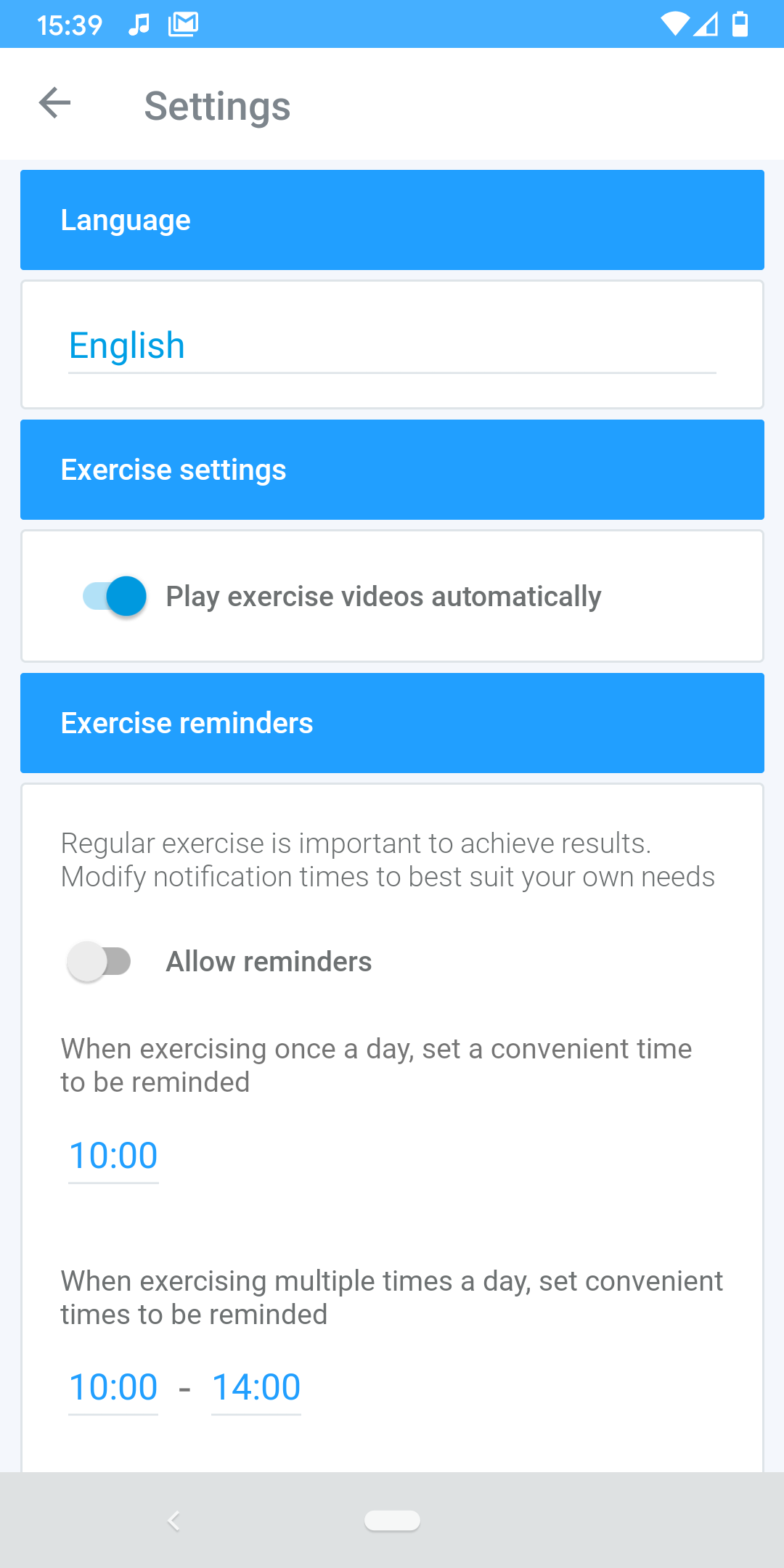A detailed screenshot of a settings page is displayed. The background is gray, while each section on the page has a white background. At the top, a light blue heading titled "Language" lists "English." Below that, the "Exercise Settings" section is also highlighted in blue. Here, users have options to:

1. **Play exercise videos automatically** – A feature indicated with a toggle switch.
2. **Exercise reminders** – An option crucial for regular exercise and achieving results, also equipped with customizable settings.

Further down, some additional options and information are provided:

- **Allow reminders**: This is shown in bold and is currently toggled off. It emphasizes the importance of setting a convenient time for reminders when exercising once a day. The set time is currently displayed as "10," highlighted in blue.
- For those exercising multiple times a day, there is a suggestion to set convenient reminder times. The example given is "10 to 1400."

At the bottom of the page, there is a gray button, completing the layout of this user-friendly and clean interface designed to help users manage their exercise routines effectively.